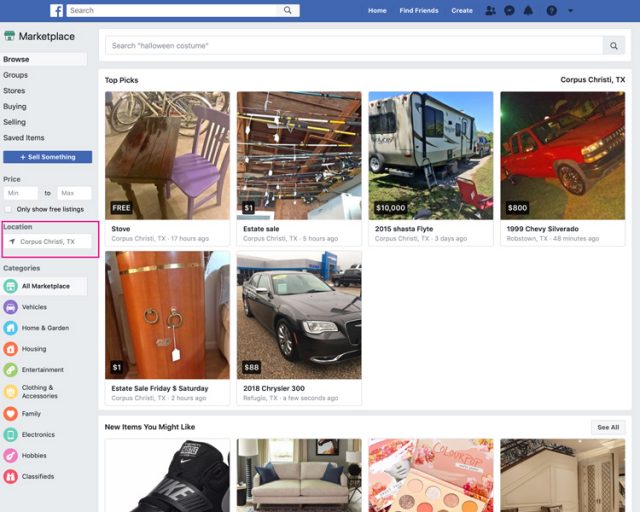Caption:
---
The image depicts a screenshot of the Facebook interface, specifically focused on the Marketplace section. At the top, there's a distinct blue bar featuring the Facebook logo, a search bar, and navigation options including "Home," "Find Friends," and "Create." Accompanying these options are several icons. 

Below the main navigation, the Marketplace section is highlighted, presenting numerous browsing options such as "Browse," "Groups," "Stores," "Buying," "Sells," and "Saved Items." A prominent blue button labeled "Sell Something" invites users to list their items for sale. A secondary search bar prompts with "Search Halloween Costume."

The main content area displays "Top Picks," showcasing various listings. Items include a stove, accompanied by a table and chair with the location marked as "Corpus Christi, Texas," posted 17 hours ago. Other listings feature fishing rods under the "Estate Sale" category, an RV priced at $10,000 (2015 Shasta Flight), a $800 1999 Chevy Silverado, a generic "Estate Sale Friday Saturday" entry for $1, and a $88, 2018 Chrysler 300.

Below the main listings, there are "New items you might like," which include a couch, makeup, Nike merchandise, and what appears to be the interior of a house. On the left side of the screen, a highlighted location box with a purple shade is visible, followed by various categories such as "Vehicles," "Home and Gardens," "Housing," "Entertainment," and more.